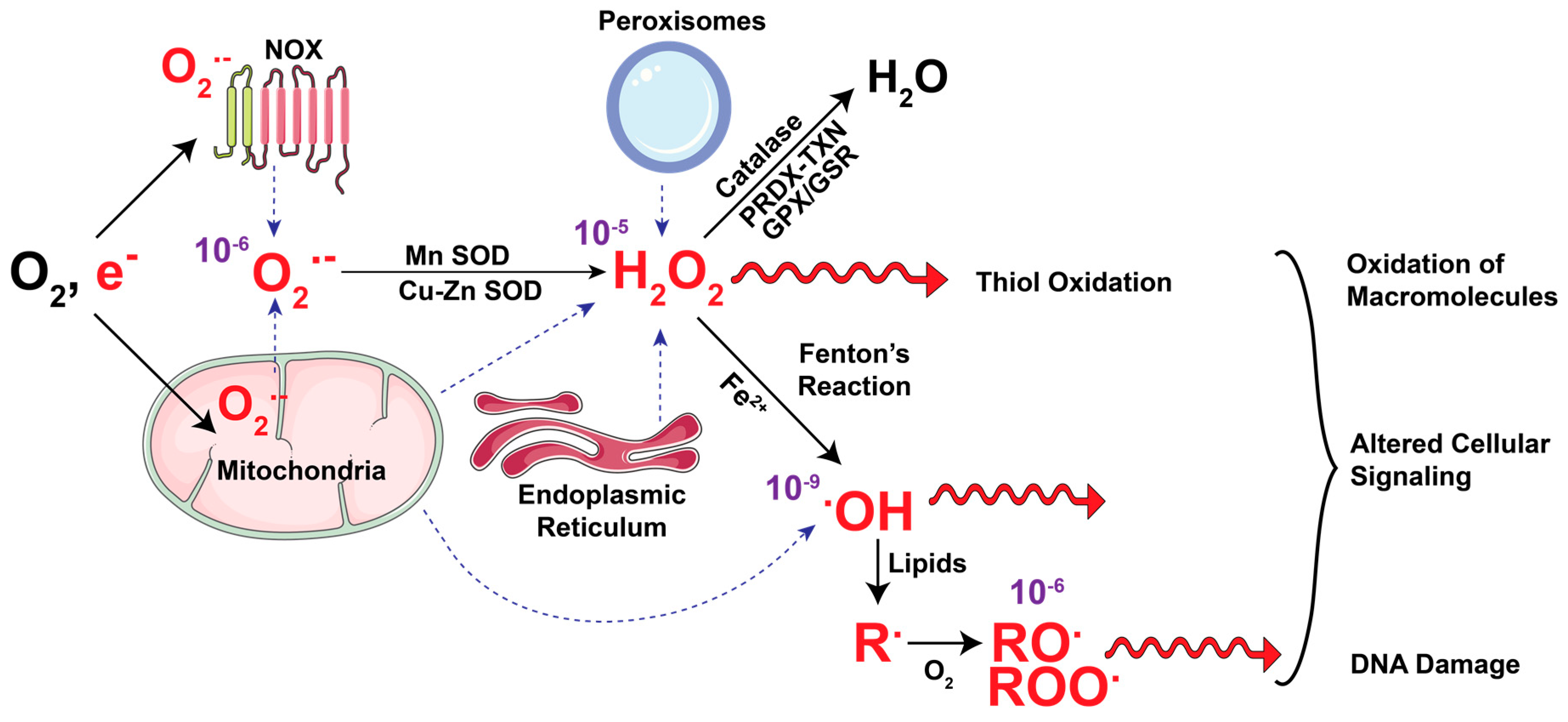The image depicts a detailed diagram of a biochemical process focused on oxygen metabolism and its impacts on cellular components. Starting from the left, the diagram begins with molecular oxygen (O2), represented with black arrows pointing towards mitochondria and possibly a depiction of DNA in green and red. Notations on the diagram include "NOX" (NADPH oxidase), which further drives the process with arrows pointing from left to right, illustrating the transformation of O2 into hydrogen peroxide (H2O2).

Various cellular structures are involved, such as the endoplasmic reticulum and peroxisomes, shown in blue circles, which interact with H2O2. The H2O2 then undergoes decomposition via catalase, releasing water (H2O), as well as through the action of other enzymes like PRDX, TXN, GPX, and GSR, delineated by arrows. Another pathway shown is the Fenton reaction, catalyzed by Fe2+, resulting in the production of hydroxyl radicals (OH), which target lipids, transforming them into reactive oxygen species (RO and ROO).

Consequent arrows indicate downstream effects such as DNA damage, altered cellular signaling, and oxidation of macromolecules. The diagram is well-annotated, with red lettering at various critical points, and arrows clarifying the sequence of chemical reactions and interactions, summarizing complex biochemical pathways and their implications in cellular damage and oxidative stress.